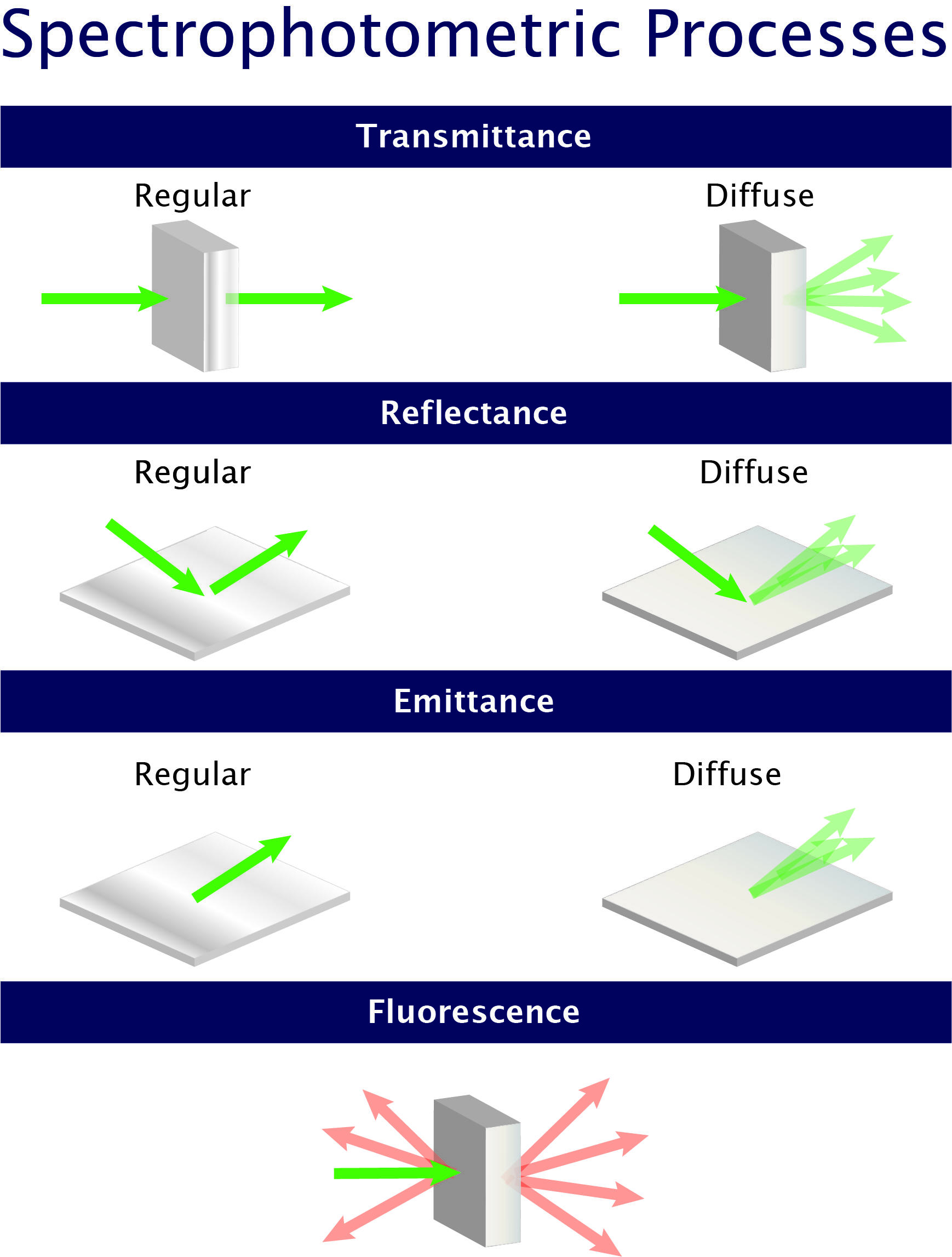The image is a detailed spectrophotometric diagram on a white background, structured with blue bars across four main sections - Transmittance, Reflectance, Emittance, and Fluorescence. Each section is further divided into two subcategories: Regular and Diffuse. 

Under Transmittance, green arrows illustrate the path of light, with regular transmittance showing a straightforward arrow passing through a block, while diffuse transmittance features multiple arrows spreading out. Reflectance follows a similar pattern, where regular reflectance is depicted with a single green arrow bouncing back and diffuse reflectance shows several arrows scattering in various directions. Emittance, too, differentiates with a singular green arrow for regular emittance and multiple diverging arrows for diffuse emittance.

Fluorescence, distinct from the others, uses red arrows instead of green. Here, a single green arrow enters the block, and multiple red arrows emanate in both directions from the block, resembling an explosive dispersal. Each descriptive label is styled with white lettering on a blue background for clear categorization, and overall, the diagram visually emphasizes the complexity and divergent paths of light in diverse spectrophotometric processes.